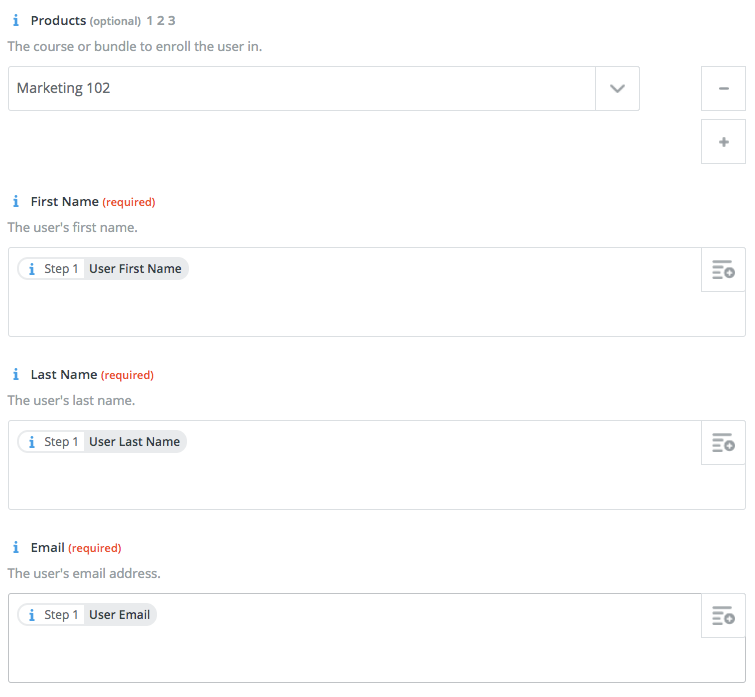Screenshot of a Website's Enrollment Form

The screenshot captures a segment of a website, featuring an enrollment form. In the top left corner, the header "Products Optional" is prominently displayed. Directly beneath this, the form is labeled to guide the user on the specific course or bundle they can enroll in, with "Marketing 102" clearly listed.

The form itself is a straightforward contact page requiring users to provide basic information. The fields are marked as required in bold red text, indicating the necessity of their completion. The required entries include:
- **First Name**: A field for the user's first name.
- **Last Name**: A field for the user's last name.
- **Email**: A field for the user's email address.

Notably, the input boxes for these details are unusually large, providing excessive space that visually suggests each entry could accommodate a paragraph, despite the requirement being just a single word or a short phrase, such as a name or an email address. This disproportionate design appears cumbersome and inefficient for the simplistic nature of the data being collected.

Overall, the captured form appears to be a basic information entry page, albeit with a somewhat clunky layout.